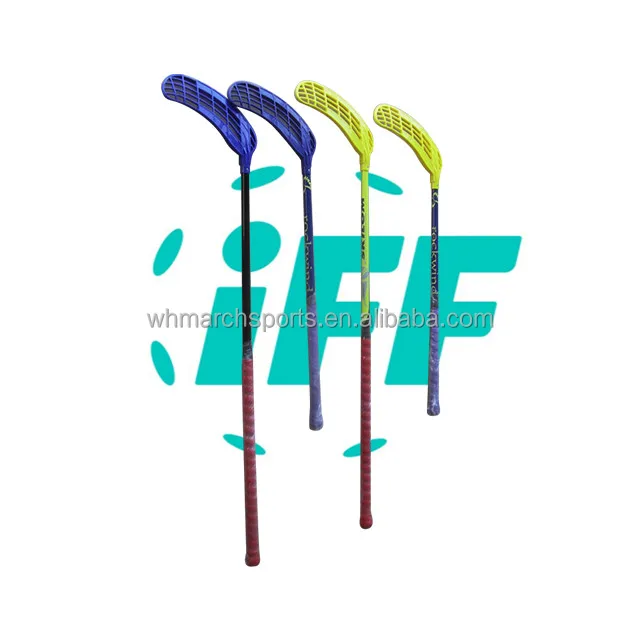The image features four sport sticks, resembling field hockey sticks, arranged in a row against a plain white background. The handles of the sticks are oriented at the bottom of the image, with the curved heads at the top. The sticks vary in length, with alternating sizes—long, short, long, and short. The two sticks on the left have blue heads and grips, while the two on the right have yellow heads and grips.

The stick on the far left has a red grip, a black handle, and a blue head. The stick next to it, slightly behind to the right, also has a blue head and grip with a black handle. Moving further right, the third stick has a red grip, a yellow handle, and head. The stick on the far right, slightly further back, features a blue grip, black handle, and a yellow head.

Dominating the background is a teal-colored logo with a lowercase "i" followed by two uppercase "F"s, surrounded by teal circles. Additionally, a watermark is visible in light gray across the center of the image, reading "WHMARCHSPORTS.EN.ALIBABA.COM." The overall image is bright, clear, and well-lit, showcasing the sticks in crisp detail.